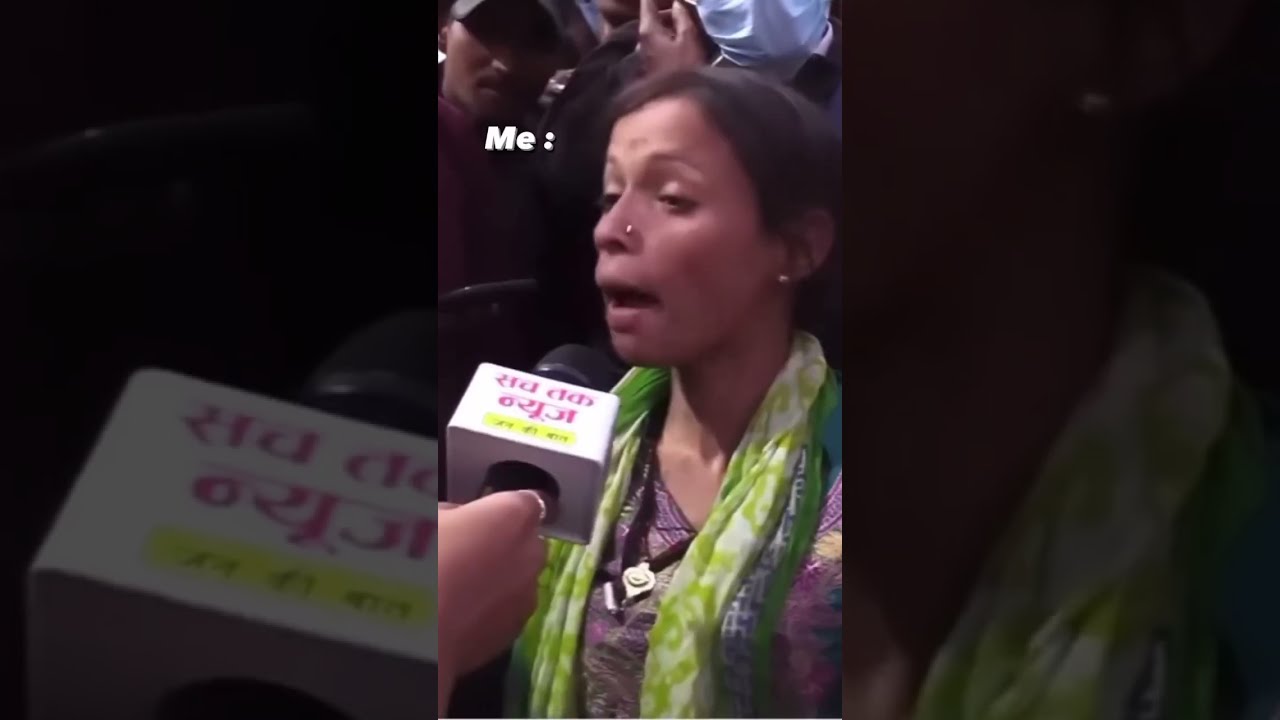In this image, which appears to be a still from a video, a woman is seen addressing a microphone held close to her face, possibly at a protest or public event. She has long, dark hair pulled back, a nose ring, and stud earrings. Her skin is brown, and she's wearing an intricate purple and white blouse with a green scarf draped around her neck. The black microphone with a white rectangular handle, inscribed with text in what looks like Arabic script, is being held by another person with brown skin. Despite the image's slight blur, the woman’s passionate expression is evident as she speaks. A sea of people is visible in the background, suggesting a crowded event with onlookers. The word "ME" is captioned on the top left of the image.